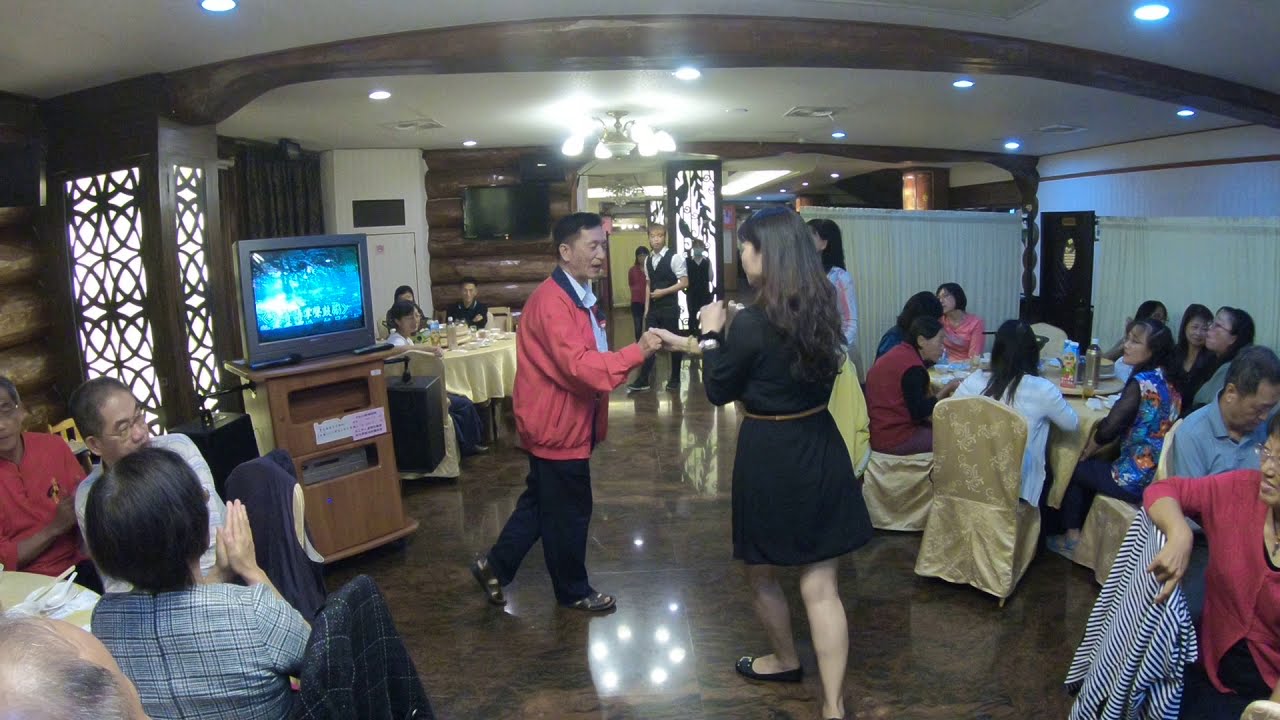In the image, a festive scene is set in what appears to be a restaurant or banquet hall with shiny brown floors and a low white ceiling adorned with a chandelier and recessed lighting. Prominent in the center is a man, an older gentleman in a red jacket, black pants, and sandals, dancing with a woman wearing a black dress and black shoes. They are holding hands in a dance position. The woman has long, wavy hair and is not facing the camera.

Surrounding the dance floor are round tables covered with yellow tablecloths and seated guests on chairs adorned with yellowish mustard-colored covers. The tables are cluttered with plates and party items, indicating an ongoing celebration. Guests are dressed in a mix of casual and formal attire, with some men in nice shirts and women in dresses or sweaters. Most of the attendees appear to be of Asian descent.

On the left side, in between the tables, is an old-fashioned TV, possibly a karaoke machine, with a blue screen and a microphone. Behind this TV is a lattice-like window, and to the right of it, another table with people. In the background, a waiter in a black vest is seen observing the dancers. The setting exudes an atmosphere of joy and celebration, as groups of people are both mingling and watching the dancing couple, enhancing the lively ambiance of the scene.